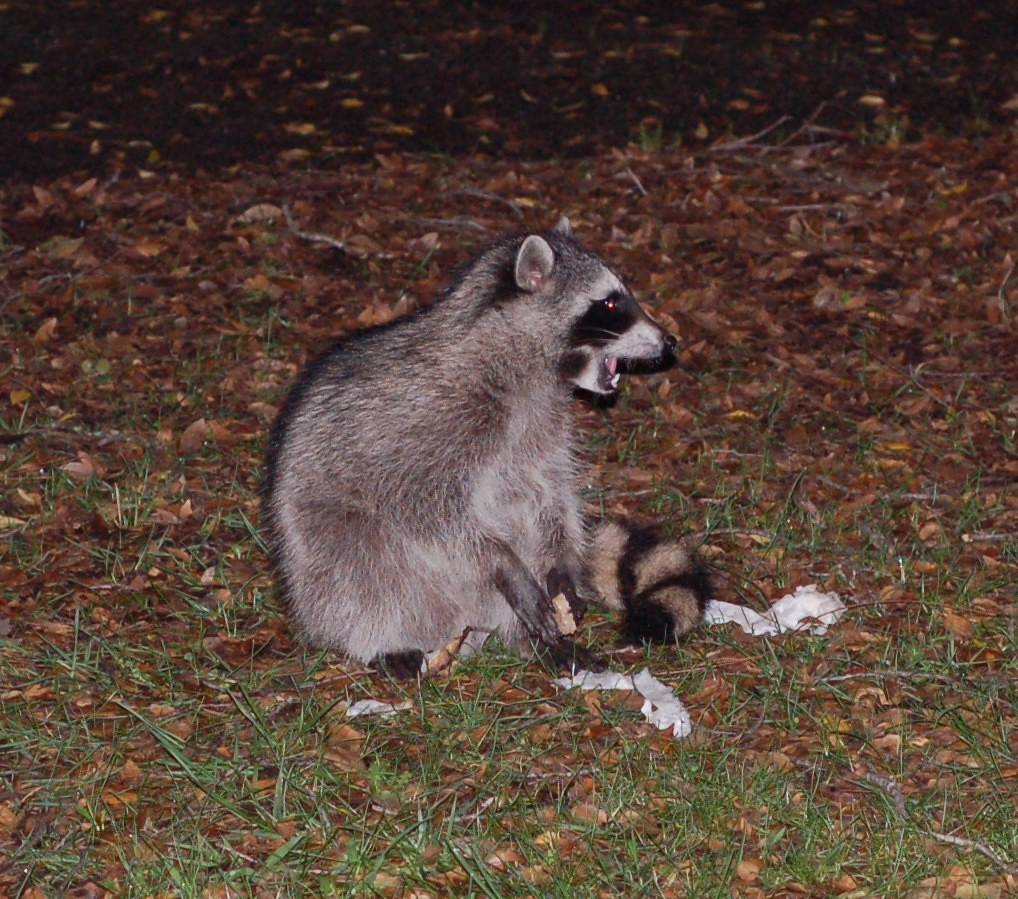Captured in the stillness of a nighttime setting, this nature photograph, taken with a flash, reveals a lively scene amidst the darkness. The ground is blanketed in a thick carpet of brown leaves, interspersed with vibrant green blades of grass. Center stage is a raccoon, caught in mid-chew, its gaze directed to the right. The raccoon's distinctive features are clearly visible: its gray fur is accentuated by a black mask and a white muzzle, and its bushy tail, coiled around its body, shows off the familiar brown and black stripes. Scattered bits of trash around the raccoon hint at its foraging habits, adding a touch of poignancy to this glimpse of urban wildlife.